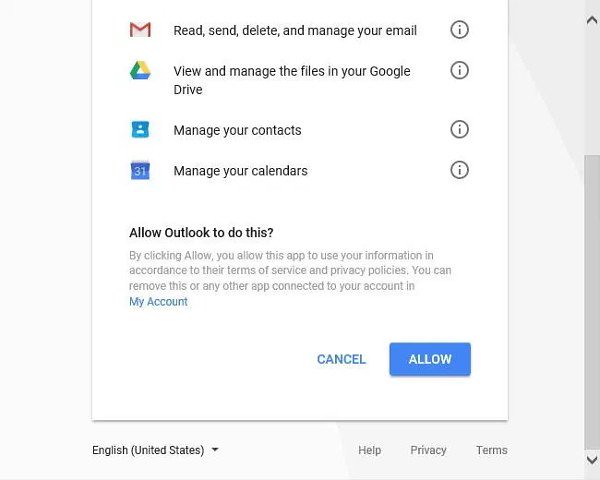The image depicts a permissions request page from Outlook against a white background. The header includes a series of icons representing various services and the permissions they require:

1. At the top left, the Gmail symbol appears, followed by text in black that states, "Read, send, delete, and manage your email."
2. Beneath the Gmail section, the Google Drive symbol is shown with accompanying text that says, "View and manage the files in your Google Drive."
3. Further below, a contact symbol is displayed with the text, "Manage your contacts" next to it.
4. A calendar symbol is situated below the contact symbol, with the text, "Manage your calendars" adjacent.

Below these icons and descriptions, the page features a prompt: "Allow Outlook to do this?" followed by an explanatory paragraph: "By clicking allow, you allow this app to use your information in accordance to their terms of service and privacy policies. You can remove this or any other app connected to your account in my account." 

The page offers two interactive options: a bold blue "Allow" button and a "Cancel" option. At the bottom of the panel, "English (United States)" is indicated, followed by clickable text options for "Help," "Privacy," and "Terms."